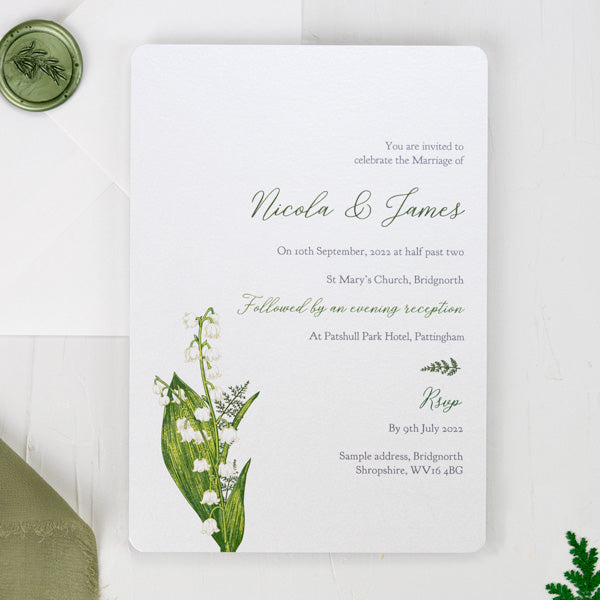The image is a color photograph in a square format, depicting a detailed, elegant wedding invitation. Centered against a white satin cloth background that mimics a white wooden table, this vertically-oriented, rectangular invitation with rounded corners features predominantly blue text. At the top, it reads, "You are invited to celebrate the marriage of," with "Marriage" capitalized for emphasis. The names, "Nicola Ensemble James," appear prominently in green cursive, followed by details in blue text: "on 10th, September, 2022, at half past two, St. Mary's Church, Bridge North." Below this, in green cursive, the invitation continues, "followed by an evening reception," and reverts to blue text for the location: "at Patchell Park Hotel, Paddingham."

The design includes botanical elements: a green leaf illustration extending to the left and stems of white baby's breath flowers against a dark green leaf background in the lower left corner. A notable element is a green wax seal with a fern illustration in the upper left. The RSVP information, "RSVP by 9th, July, 2022," along with a sample address, "Sample Address, Bridge North, Sharp Fire, WV 16, Fort Beach," appears towards the bottom. The right margin of the invitation maintains alignment, with all text well-placed and aesthetically consistent, highlighting the formal and groomed nature of the event.